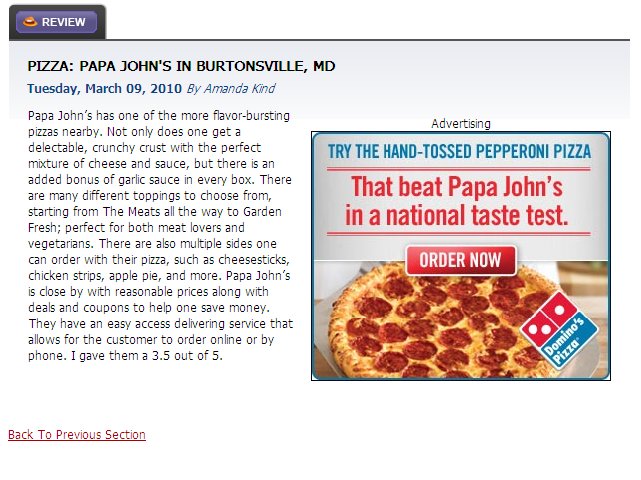This detailed review is about the Papa John's location in Burtonsville, Maryland, as featured under the "Review" tab. The review, titled "Pizza:" was written by Amanda Kind and dated Tuesday, March 9, 2010. Amanda commends Papa John's for offering one of the most flavor-packed pizzas in the area. She highlights the delectable, crunchy crust and the perfect blend of cheese and sauce in every box. Additionally, she points out that each pizza comes with a complimentary garlic sauce. Amanda mentions the variety of toppings available, catering to both meat lovers and vegetarians, ranging from various meats to garden-fresh vegetables. She also notes the availability of multiple side orders, including cheese sticks, chicken strips, apple pie, and more. Amanda concludes by appreciating the nearby location, reasonable pricing, and frequent deals and coupons that help customers save money.